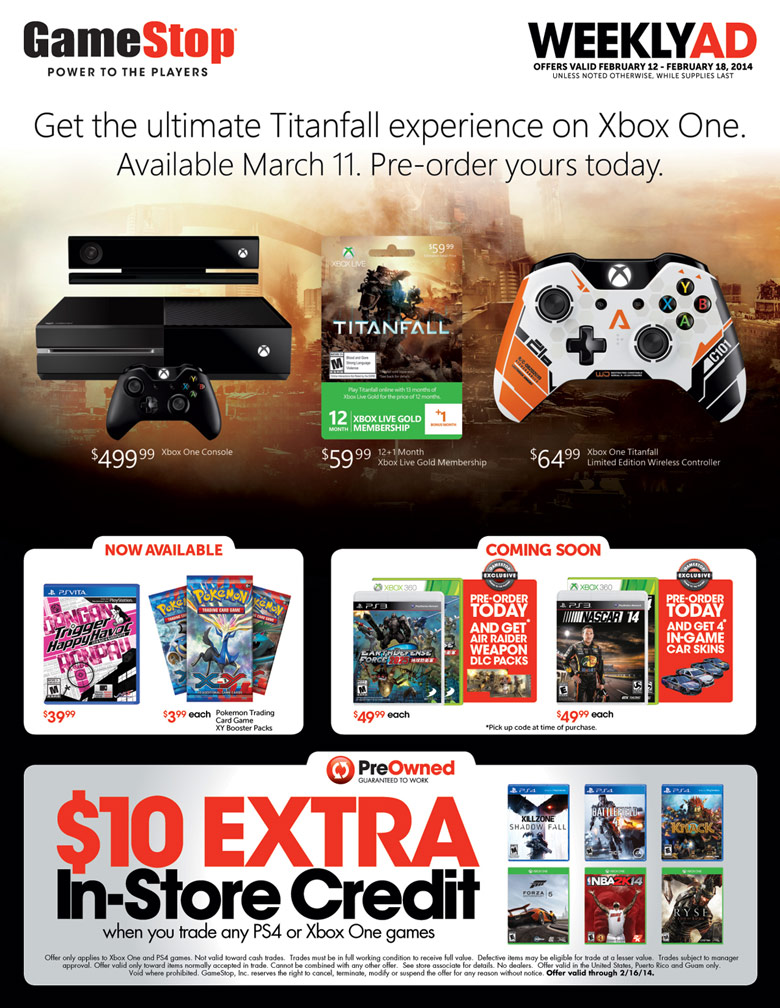**GameStop Advertisement: Ultimate Titanfall Experience**

Experience the ultimate in gaming with GameStop's exclusive promotion for Xbox One and Titanfall! This high-quality advertisement poster, designed with vibrant and engaging graphics, aims to capture the attention of gaming enthusiasts.

**Top Section:**
- **Top Left Corner:** GameStop logo with the tagline "Power to the Players."
- **Top Right Corner:** Important dates "Weekly ad offers valid February 12th through February 18th, 2014," followed by "Unless noted otherwise, while supplies last."

**Main Header:**
- Bold and eye-catching text: "Get the Ultimate Titanfall Experience on Xbox One, available March 11th, pre-order yours today."

**Highlighted Items:**
- **Xbox One Console:** Priced at $499.99
- **12-Month Xbox Live Gold Membership:** Priced at $59.99
- **Xbox One Titanfall Limited Edition Wireless Controller:** Priced at $64.99

**Device Imagery:**
- Images of the sleek Xbox One console, the membership game card, and the specialty Titanfall-themed controller enhancing the visual appeal.

**Availability Sections:**
- **Now Available:** Showcases current offerings with prices.
- **Coming Soon:** Displays upcoming items, creating anticipation with their corresponding prices.

**Pre-Owned Section:**
- **Large Highlighted Area:** "Pre-Owned, Guaranteed to Work," emphasizing value.
- **Special Offer:** "$10 extra in-store credit when you trade any PS4 or Xbox One games."

**Additional Content:**
- To the right, covers of various Xbox One and PS4 games.
- Small disclaimer text below detailing additional conditions or information.

This meticulously detailed layout ensures that customers are fully informed about the amazing deals and exclusive promotions available at GameStop!